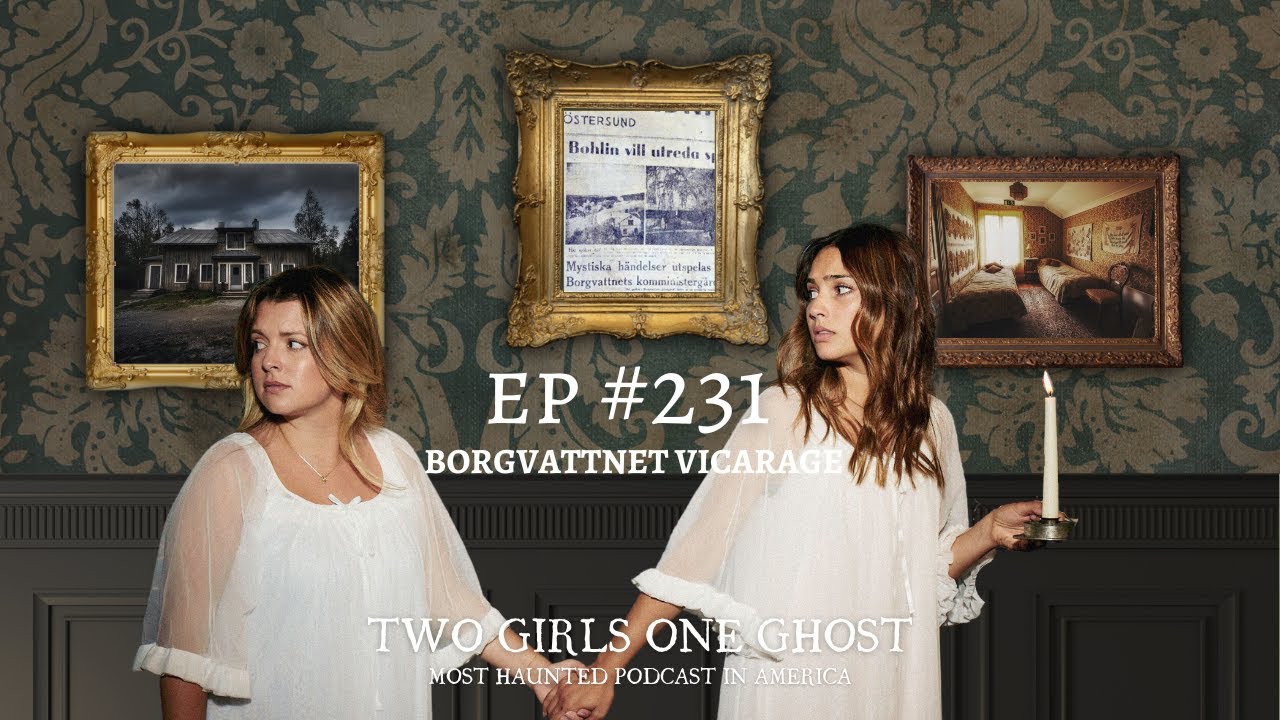This promotional image or thumbnail for the podcast "Two Girls, One Ghost," described as the "most haunted podcast in America," showcases a spooky and atmospheric theme. Set against a vintage backdrop of green and white floral wallpaper with an underlying gray wooden wall, the image features three digitally imposed photo frames. These frames contain eerie visuals: one of a haunted-looking house, another of a newspaper clipping, and the third displaying a rundown hotel room. Central to the image are two women dressed in sheer white nightgowns. The woman on the left, chubbier with brown hair and blonde highlights, and the thinner woman on the right, holding a lit candle in her left hand, both gaze fearfully to the left. Golden and brown antique-style frames border the photos, enhancing the vintage and haunting ambiance. The text overlay reads "EP No. 231, Vorfenay Vicarage," with the show title "Two Girls, One Ghost" and its tagline, "Most haunted podcast in America," prominently displayed, encapsulating the eerie essence of the episode.